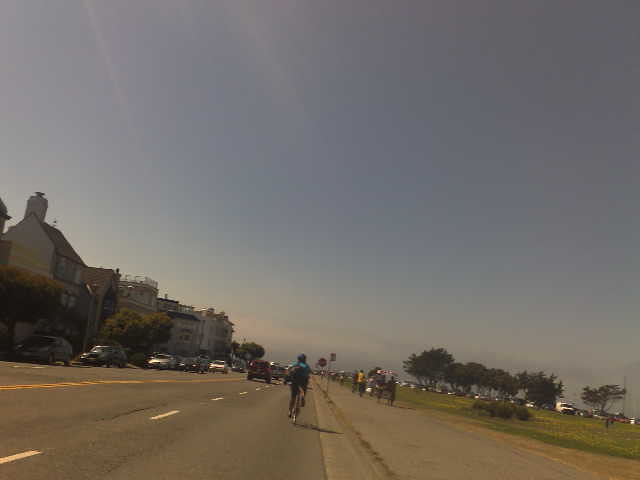A photograph captures a bustling urban street scene. In the foreground, a cyclist wearing a green top and a helmet pedals away from the camera, dominantly positioned in the center of the image. Flanking the cyclist on one side of the street, several parked cars line the curb, leading the eye towards a backdrop of three-story buildings, their facades showing signs of daily life and activity.

Across the street, a pedestrian footpath is alive with people strolling, framed by a neatly manicured green lawn that adds a touch of nature to the scene. Beyond the lawn, a line of trees creates a natural barrier before more parked cars come into view. The sky above is light blue, gradually fading into a hazy light gray at the horizon, encapsulating the city in a serene morning or evening light. Scattered cars on the road complete the dynamic tableau, contributing to the impression of a typical, lively day in the city.